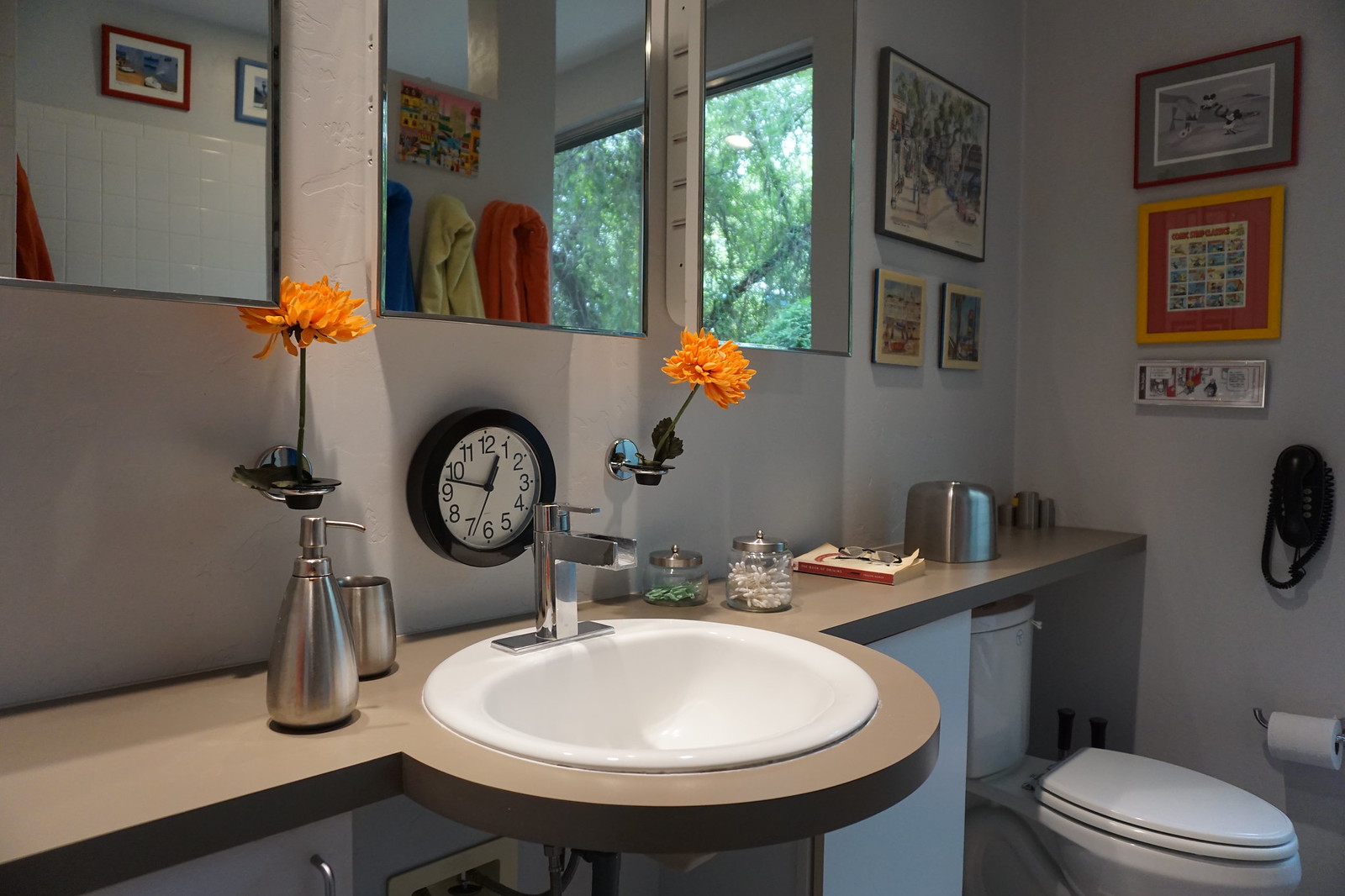The bathroom image depicts a vividly detailed interior. The scene is orchestrated with an array of mirrors and paintings that dominate the visual landscape. At the top left, center, and right of the wall, there are three mirrors, each distinctly placed to reflect different angles of the space. Complementing these mirrors are various paintings: one on the top, one on the left, and another on the right. On the adjacent wall to the right, a series of framed artworks includes a top painting with a bordered interior scene, a middle artwork in an orange frame with a red background and a pasted print, and a small rectangular piece resembling a comic strip.

At the bottom of the image, there's a toilet accompanied by a roll of toilet paper. An intriguing detail is the coiled cable affixed to the wall above the toilet. To the right of the toilet, a countertop in a grayish-brown hue hosts several items. A cylindrical silver container sits atop it, and further left, a book with reading glasses is carefully placed. Beside the book, a glass jar filled with Q-tips features a matching silver lid and shares the space with another unidentified jar.

Enhancing the decorative theme of the bathroom, there's a flower held up by a wall-mounted holder, showcasing a stem and bright orange leaves. Beside it, another wall holder leads to the centerpiece, a clock with hands positioned between 12 and 1, 9 and 10, and 7 and 6 respectively. Beneath this clock, a silver faucet and white porcelain sink are framed by the grayish-brown countertop lip.

A silver pump soap dispenser and a matching cup are adjacent to the sink. The reflections in the mirrors reveal an arrangement of three rows in blue, yellow, and green hues and a window view to the outside world adorned with trees and green leaves. The level of detail in the photograph captures the eclectic yet harmonious design of the bathroom.